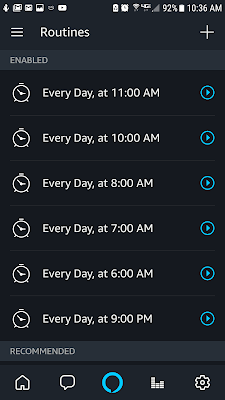A detailed screenshot taken from a mobile phone displays a variety of icons and information against a predominantly black background with white text. 

At the top left corner, there is a small animated figure, followed by a mail symbol, another mail symbol, the Instagram icon, the Amazon Prime logo, and the YouTube icon. A small black space separates these icons from the information on the right side, where we find a battery-saving symbol, an alarm icon, a diamond-shaped icon, the 4G symbol, very low cell phone coverage bars, a battery indicator showing 92% charge, and the time displayed as 10:36 AM.

Just below this top bar, there is a line with three small horizontal lines on the left side, labeled "Routines." On the right side of this line, there is a plus sign. Below this, a gray bar reads "Enabled" in gray text.

The main portion of the screenshot features six alarm settings, each marked by an alarm clock icon. The alarms are set for 11:00 AM, 10:00 AM, 8:00 AM, 7:00 AM, 6:00 AM, and 9:00 PM respectively. Each alarm setting has a blue circle with a blue arrow pointing to the right on the right side.

Towards the bottom of the screen, another gray bar displays the text "Recommended" in gray. At the very bottom, familiar icons for navigation include a home button, a speech bubble, the blue Alexa logo, a bar graph, and a gear icon.